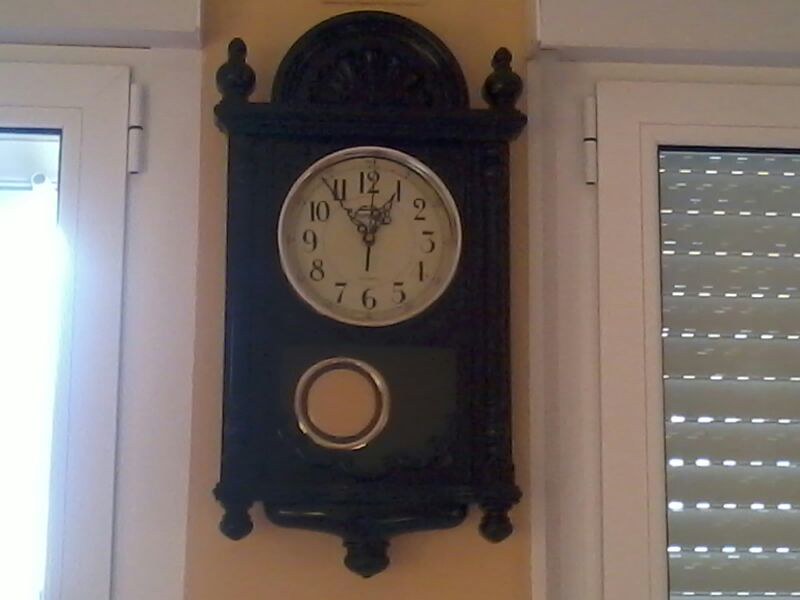A medium-sized grandfather clock is prominently displayed on a small section of wall in a hallway, nestled between two doors. The clock features a circular face with traditional digits from 1 to 12, all set against a white background, enhanced by a silver trim and sleek hour, minute, and second hands. The ornate wooden frame of the grandfather clock is further accentuated with intricate pinnacle details at both the top and bottom. Designed in a rectangular shape, the frame also includes a circular top. A brass pendulum, visible through a clear glass panel on the front, adds to the classic charm of the piece. The clock is mounted on a cream-colored wall, flanked on either side by glass doors. The door on the right is adorned with a pulled-down Venetian blind, while the door on the left allows sunlight to stream through, casting a warm glow in the hallway.